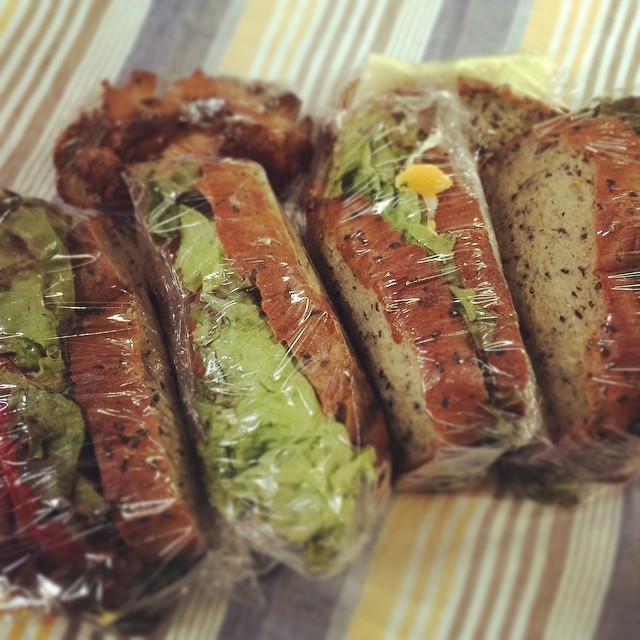The image showcases four tightly wrapped sandwiches placed in a row on a striped tablecloth. The sandwiches appear to be filled with a thick green mixture, likely avocado, based on their color and texture. One of the sandwiches, however, seems to deviate from the others and might contain lettuce and possibly eggs. The bread used for these sandwiches is a hearty, grainy type with visible seeds, resembling a mix of wheat and pumpernickel. The sandwiches are wrapped in saran wrap and sit on a tablecloth adorned with vertical stripes in yellow, white, dark brown, and touches of blue, adding a vibrant background to the setting.